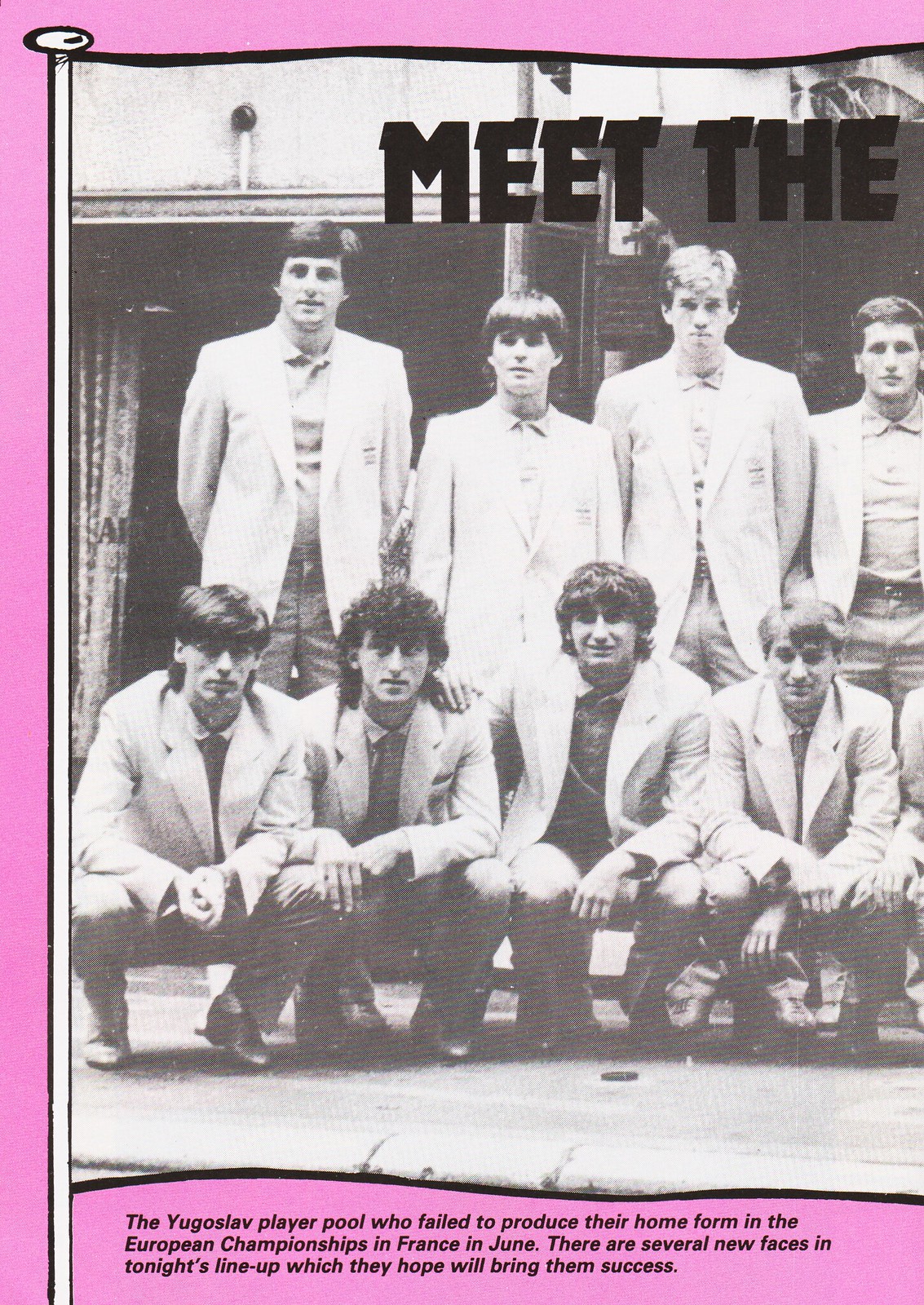This is a vintage photograph or possibly a scan of a football program, with the left side of a two-page spread cut off, leaving the right side visible. The program has a pinkish-purple background that forms an unfurling flag shape, including a topmost flagstaff. Overlaid in bold black letters is the partial title "Meet the," with the rest presumably cut off. The image features eight young men, comprising four standing in the back and four squatting in the front. They don sport coats, slacks, and shirts, some buttoned up to the top, reflecting a 60s style with longer hair. Behind them stands a building and a curtained doorway. At the bottom, in smaller black text, it reads: "The Yugoslav player pool who failed to produce their home form in the European Championships in France in June. There are several new faces in tonight's lineup which they hope will bring them success."